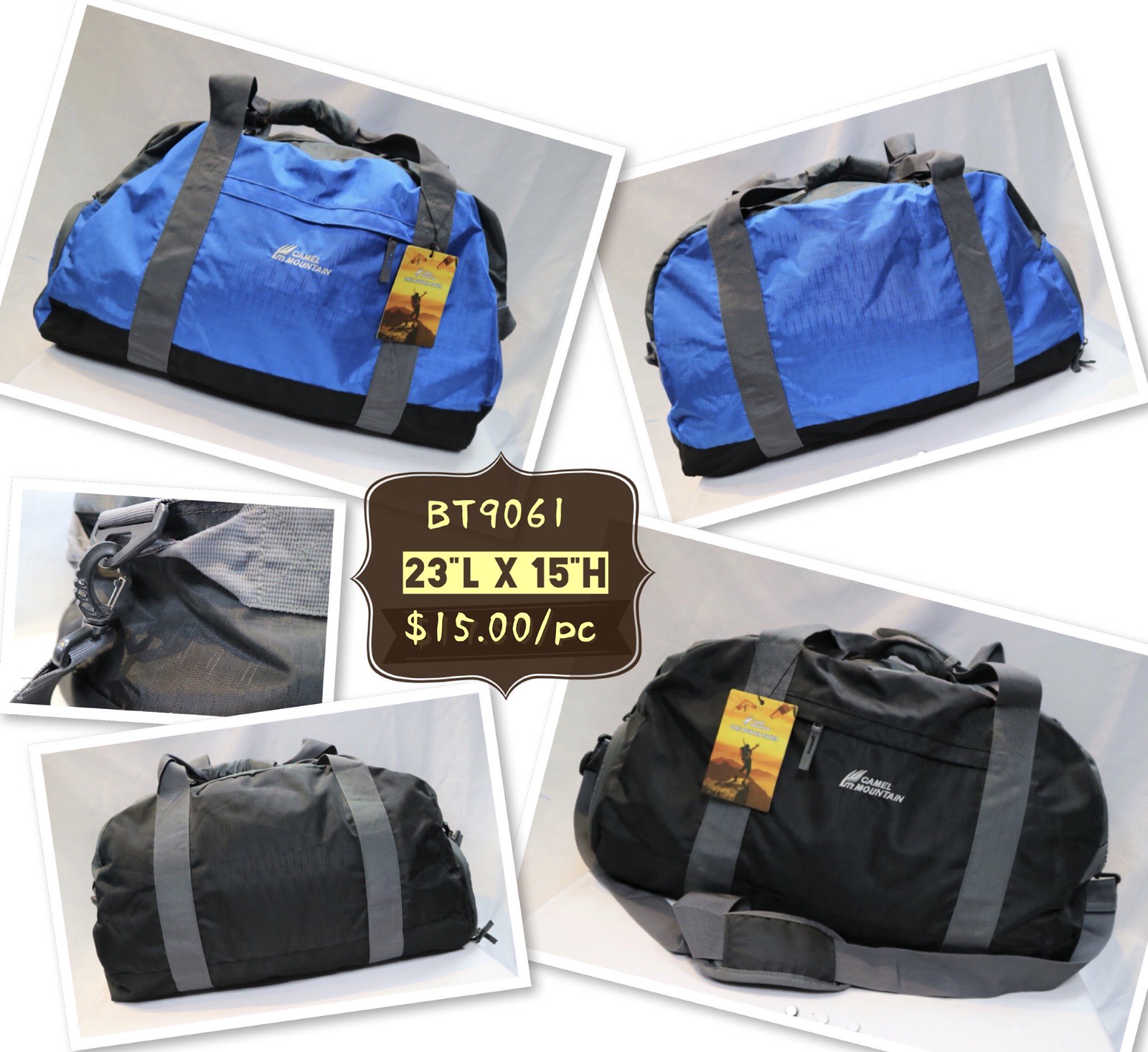The image portrays a magazine advertisement for a sporty travel duffel bag. This ad is composed as a collage of five distinct pictures, with each image housed within its own square, arranged around a central piece. The central piece features a product identifier (BT9061), the bag’s dimensions (23 inches in length and 15 inches in height), and its price ($15 each). The top two images showcase the bag in blue, depicting both the front and back views, while the two on the bottom display a black version of the bag from similar angles. A close-up shot of the clasp holding the handle to the bag occupies the middle position among the peripheral images. The duffel bags come with either black webbing (for the blue version) or gray webbing (for the black version) and feature both carrying handles and an over-the-shoulder strap, emphasizing their versatility and sporty design. The background elements incorporate a brown base with a yellow sub-background and matching brown text, though the brand name remains indistinct.